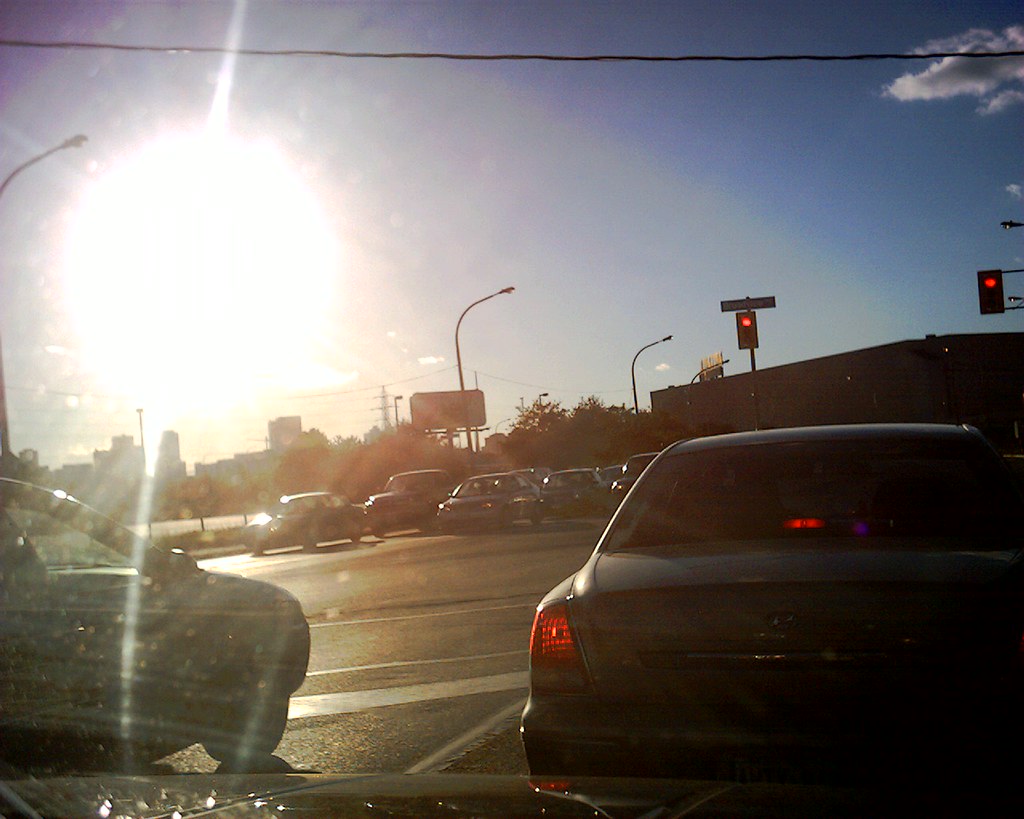This image, a square color photograph, captures a parking lot and street scene from a first-person perspective inside a stopped car. The most striking feature is the sun in the upper left-hand corner, creating a bright, glaring effect that partially obscures the frame. A prominent sunray effect, coupled with a faint rainbow arc, dominates the sky, which is mostly clear apart from a small cloud in the top right.

Visible through the windshield, a wire stretches horizontally across the scene, enhancing the urban aesthetic. The dashboard is subtly visible at the bottom edge. The lower right-hand corner of the image shows the rear of a silver vehicle, while another car appears to the left. In the background, there are two traffic lights—one positioned in the right middle and another slightly more to the left—along with a horizontal street sign, suggesting a location in the United States. The background also features a small building, a few streetlights, a billboard, and several cars dispersed throughout the scene, amounting to eight in total. Trees and additional buildings are further visible in the background, adding layers of depth and context to the image.